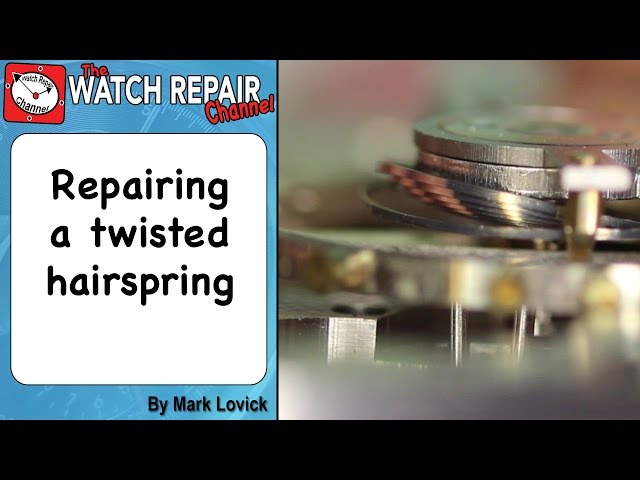The image is a color photograph, presented in a square format, and heavily detailed to serve as a thumbnail for a video titled "Repairing a Twisted Hairspring" by Mark Lovick. The right side of the image features a highly zoomed-in, representational close-up of a silver watch mechanism, focusing on a flat, silver disc with several smaller discs on top of it, and other watch parts slightly out of focus. The intricate details of the watch components are sharply rendered in a style combining photographic realism with graphic design elements.

The left side of the thumbnail is dominated by a blue vertical panel featuring multiple textual and design elements. At the top, white text reads "The Watch Repair Channel" across the blue background. Just below this, a red clock logo with a white face includes the text "Watch Repair Channel" around its top edge. Beneath this, a rounded white square with black text centers the title "Repairing a Twisted Hairspring." At the bottom of the blue panel, black text credits the tutorial to "Mark Lovick." The background is a blend of red and green irregular shapes, creating a vibrant, multicolored setting that is slightly out of focus. A horizontal black band runs along both the top and bottom edges of the image, framing the composition.